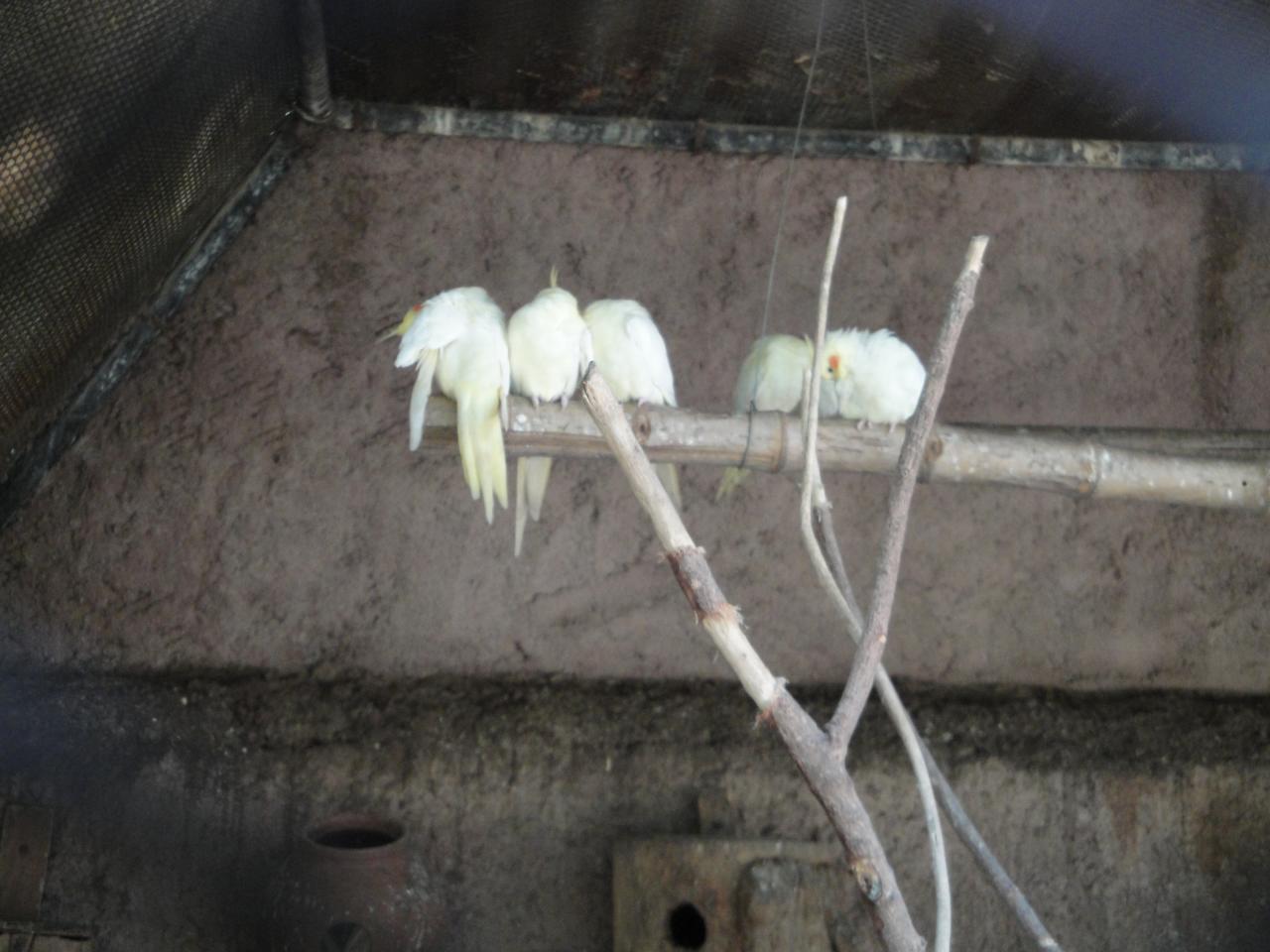The photograph captures five large white birds perched on a Y-shaped branch within a zoo enclosure. The main roosting pole is thick, bamboo-like, and light grayish-brown, intersected by a thinner branch. These branches are supported by additional sticks and wires, emphasizing the makeshift yet sturdy structure. The birds, with their white feathers cascading down and one bearing a red beak, are centrally positioned in the image. Most are facing away from the camera, except for one turning slightly towards the photographer, hinting at their varied attention. The backdrop features a gray cement wall and a black wire cage on the top left, suggesting the birds are in a confined habitat, and possibly observed by a zookeeper. The overall style of the image is a detailed photograph, capturing the serene but constrained environment of the birds.